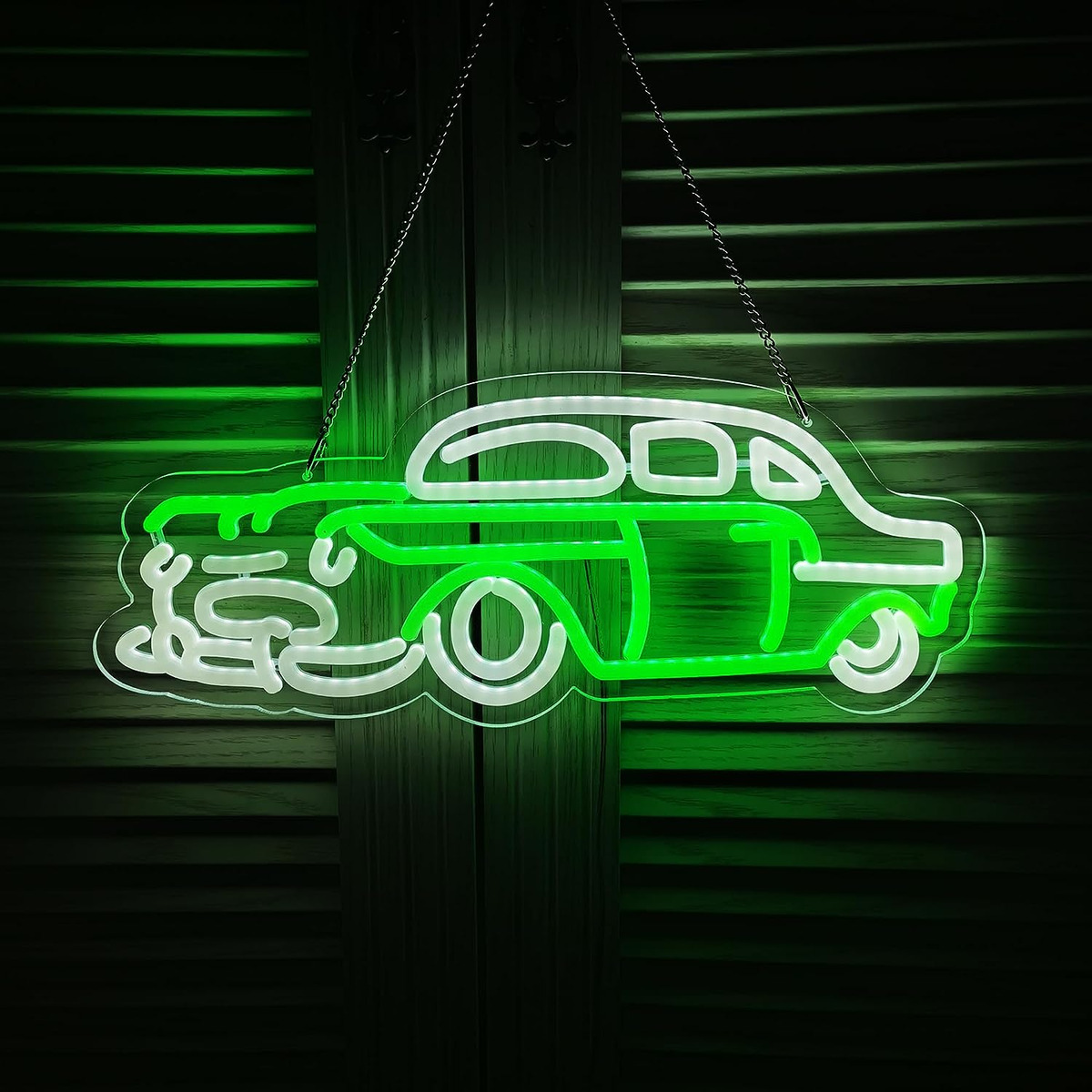This photograph, taken indoors, showcases a captivating vintage car sign made from a flat piece of clear plastic or resin, cut out in the distinct shape of an old-school car. This sign is illuminated with white and green LED-like lights, with white tubing artfully outlining the car's body, bumper, grille, headlights, wheels, windows, and doors, and green tubing accentuating the side of the car and the hood above the headlights. The sign is suspended from the top center by two small metal chains that are linked together, hanging against fully closed wooden shutters with horizontal slats about a quarter-inch wide and vertical connecting pieces that are each about half an inch wide. The glowing green lights cast a vibrant green hue across the brown wood of the shutters, intensifying towards the center and fading to black at the edges. This setting creates a striking contrast, illuminating the fine details of the shutters while highlighting the intricate design of the vintage car against the wooden backdrop.